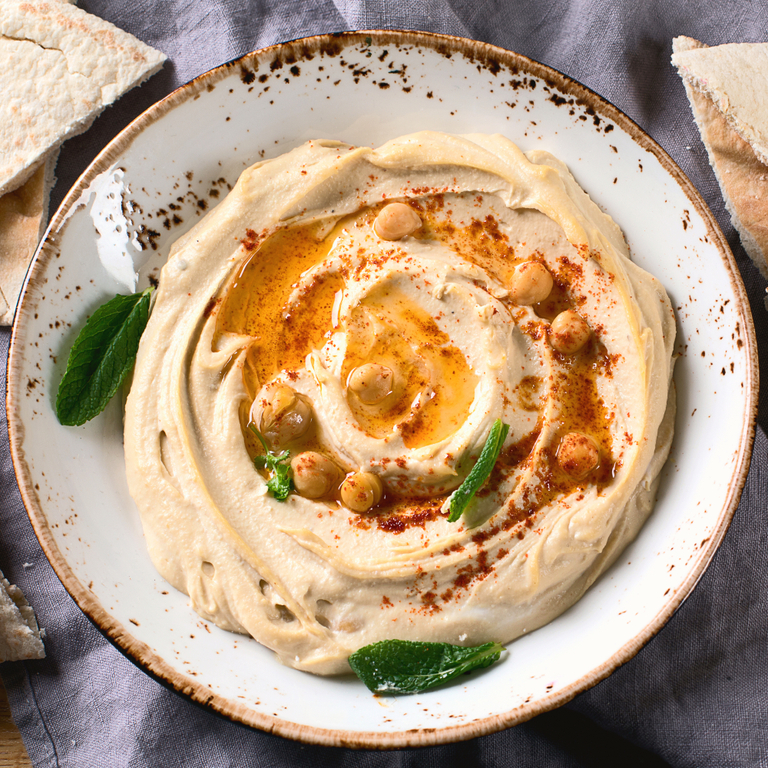This close-up photograph captures a beautifully presented serving of hummus, meticulously whipped into a circular pattern on a distinctive white ceramic plate, speckled with dark brown and copper hues, and accented by a copper rim. The hummus is garnished with pine nuts and several parsley leaves, with a drizzle of olive oil and a hint of pepper sauce adding a slight orangey color to the top. The plate is set on a blue tablecloth, further enhancing its visual appeal. Additionally, slices of pita bread, cut in half, are arranged around the plate, emphasizing the artistic and appetizing presentation reminiscent of a restaurant-quality dish.